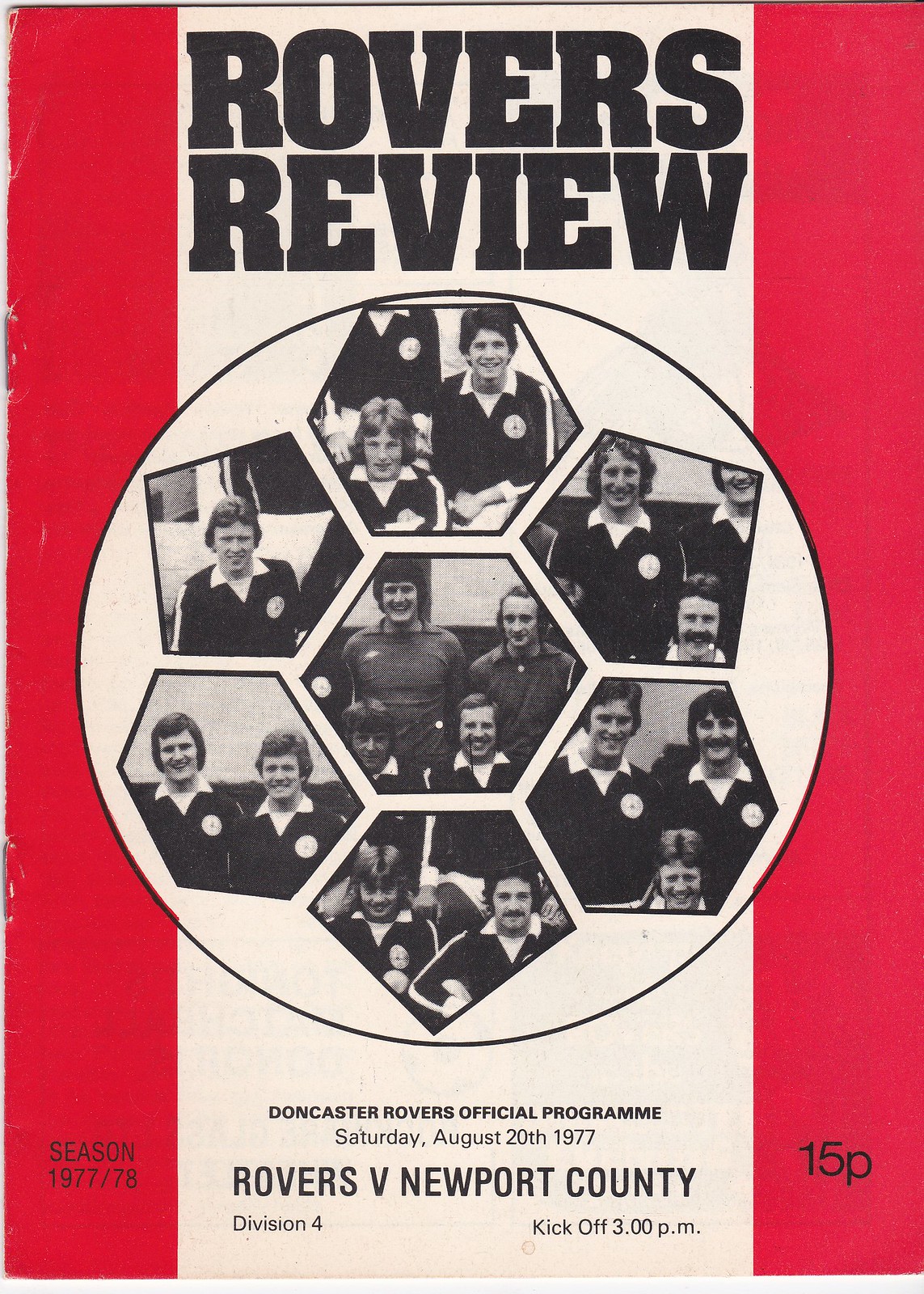The image is a cover of a vintage sports program, designed with a vertically oriented rectangular layout. The background features a cream-colored middle section flanked by two thinner vertical red stripes on either side. At the top center of the cream section, the title "ROVERS REVIEW" stands out in bold, black, block letters.

Beneath the title, a large white circle with a black outline contains seven hexagonal photographs of soccer players, who appear to be men in their 20s to 30s, all wearing uniforms with collars. The players are likely members of the Doncaster Rovers soccer team.

Below the circle, centered on the cream background, black text reads: "DONCASTER ROVERS OFFICIAL PROGRAM, SATURDAY, AUGUST 20TH, 1977, ROVERS VS NEWPORT COUNTY, DIVISION 4, KICKOFF 3 P.M." To the left of this text, on the red background, it states "SEASON 1977/78" in black print. On the right side, also on the red background, it indicates the price: "15P." This detailed design encapsulates the essence of a historic soccer program cover.